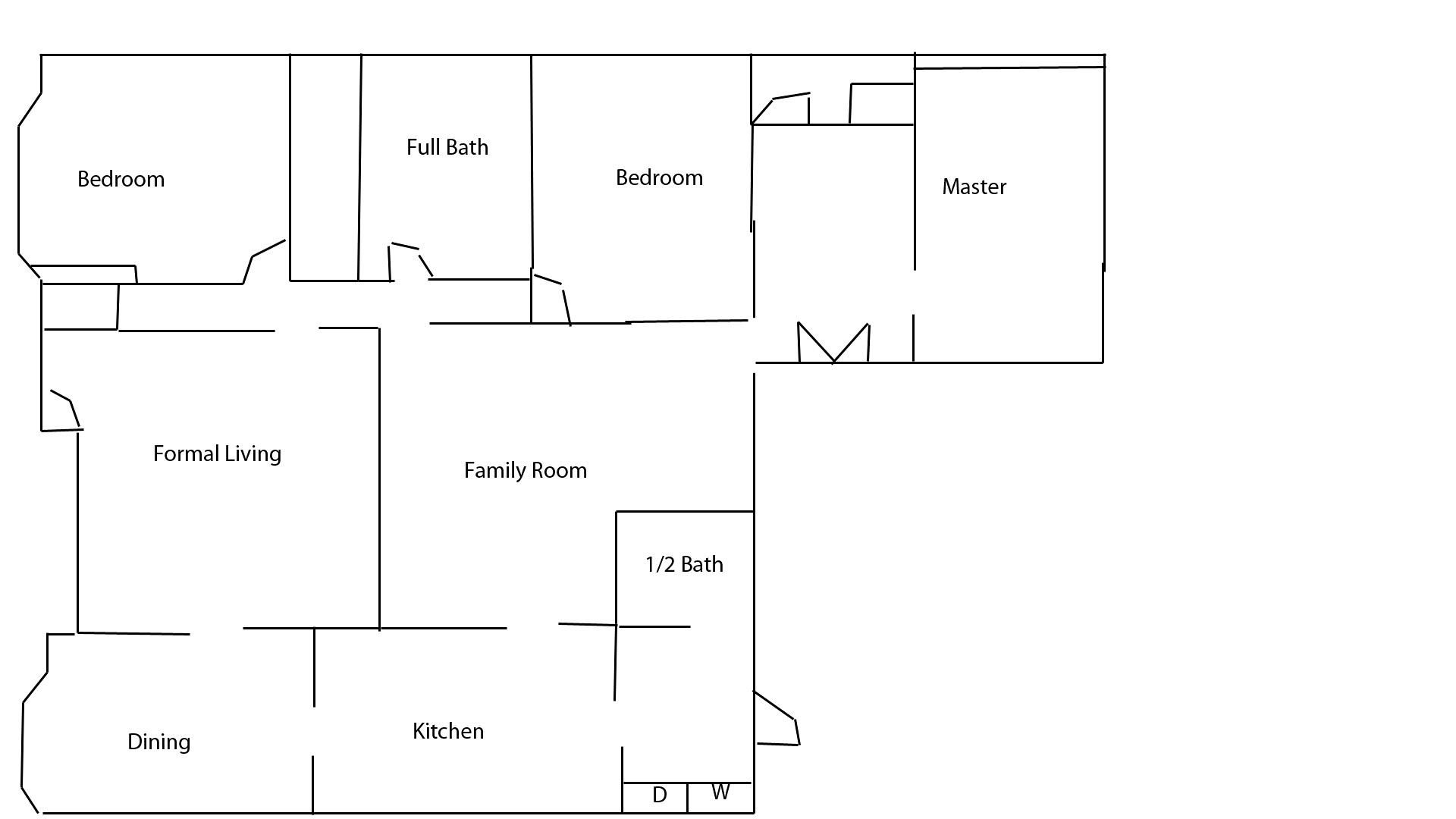This digital illustration depicts a detailed blueprint of a single-story house, showcasing the layout of various rooms and their intended purposes. The house consists of a clear arrangement of spaces, including two standard bedrooms situated between a full bathroom and a master bedroom located towards the right side. The design features both a formal living room and a family room, which are the largest rooms in the house. A half bathroom is strategically placed, partially within the family room and offering additional storage space for the adjacent kitchen.

The kitchen itself is connected to this half bath and is accessible through a corner corridor. Adjacent to the kitchen, in the bottom left corner of the blueprint, the dining room is outlined. The floor plan highlights the interconnectedness of the rooms, with numerous doors linking the family room, kitchen, hallways, bathrooms, and the dining room, ensuring a seamless and functional flow throughout the home.